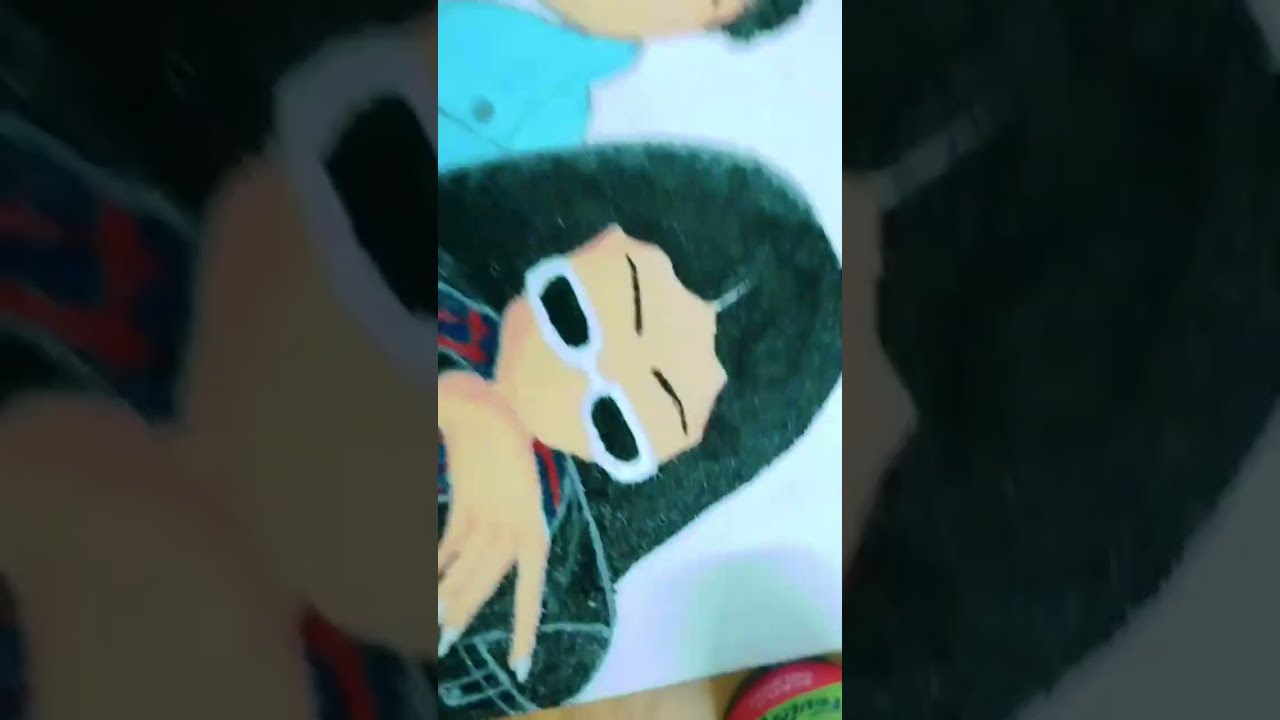The image is a vertical, cell phone-style photograph or graphical design depicting a close-up of a cartoon-like animated woman with simplified features. She has very thick, dark African-American looking hair parted down the middle, and her heavily penciled, thin eyebrows are raised high on her forehead. She wears rectangular white-framed sunglasses positioned unusually low on her face, obscuring her eyes but clearly showing her Caucasian skin. The woman has no nose or mouth, and rests her chin on the base of her right wrist, with her fingernails painted a pale blue color. She is dressed in a flannel jacket. Positioned almost 90 degrees to the right relative to the camera, she stands next to another animated character, a man with short black hair and Caucasian skin, who wears a bright blue jacket. The background of the image consists of faded, zoomed-in versions of the central picture, adding a darker, shadowy effect to the overall composition.